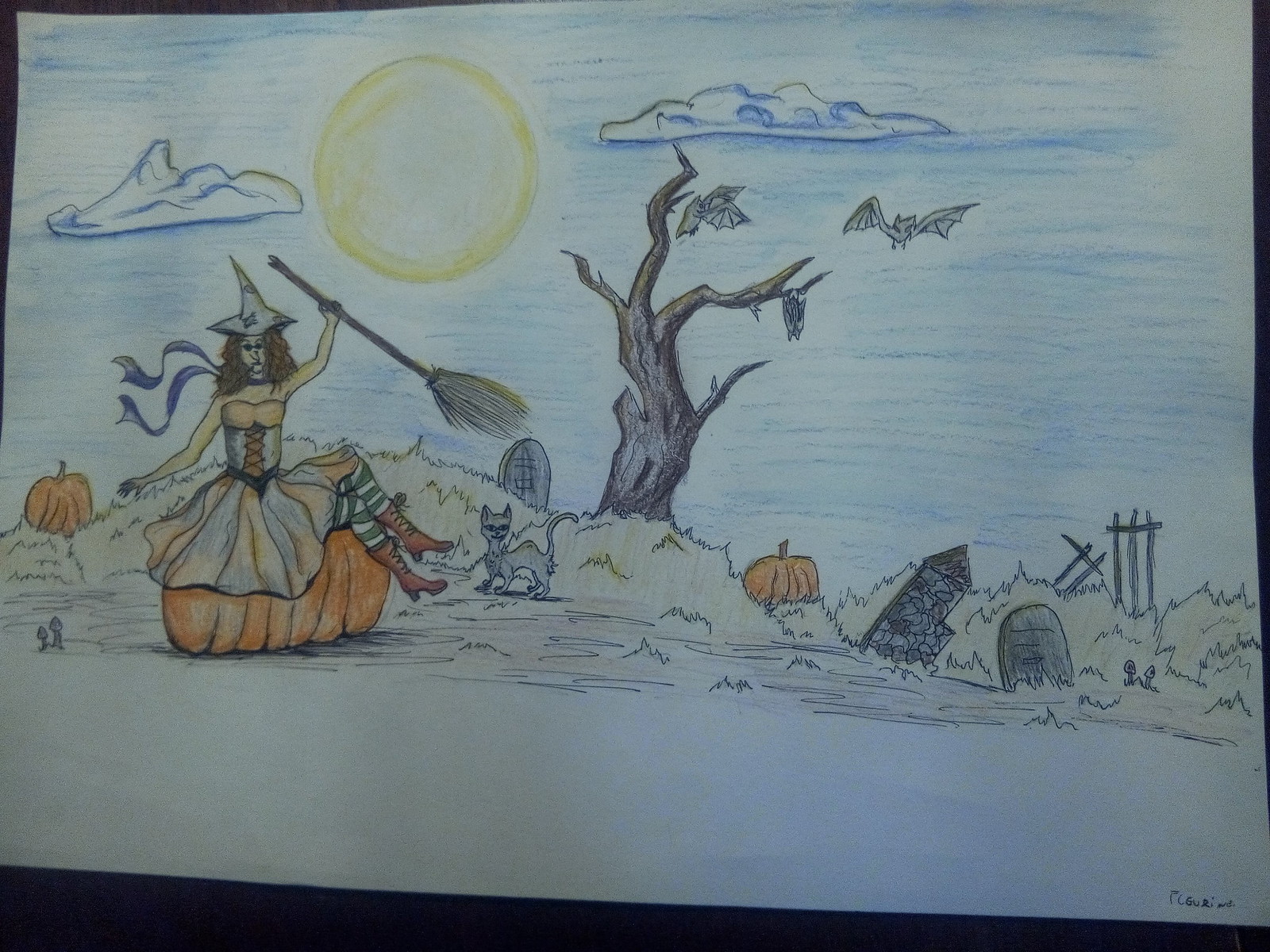This hand-drawn Halloween-themed image features a seductive witch figure sitting gracefully atop a giant orange pumpkin. She is adorned in a skirt comprising shades of white, gray, and orange, complemented by a corset-style top in light gray, black, and orange hues. Her light gray witch hat, decorated with various icons, rests stylishly on her head, and a purplish scarf drapes around her neck. The witch is holding a thin brown broom with light brown bristles, creating an air of enchantment.

Above her head, a luminous moon peers through scattered clouds. In the background, a sinister, emaciated-looking zombie cat, with a menacing expression, stands near another pumpkin. A barren brown tree, accented by two gray bats—one circling and the other hanging upside down—adds to the eerie atmosphere. The scene is further completed with tombstones in shades of gray and black, overgrown grass, and pieces of a rickety fence, all contributing to the haunted setting. At the bottom of the image, the artist's signature is discreetly placed.